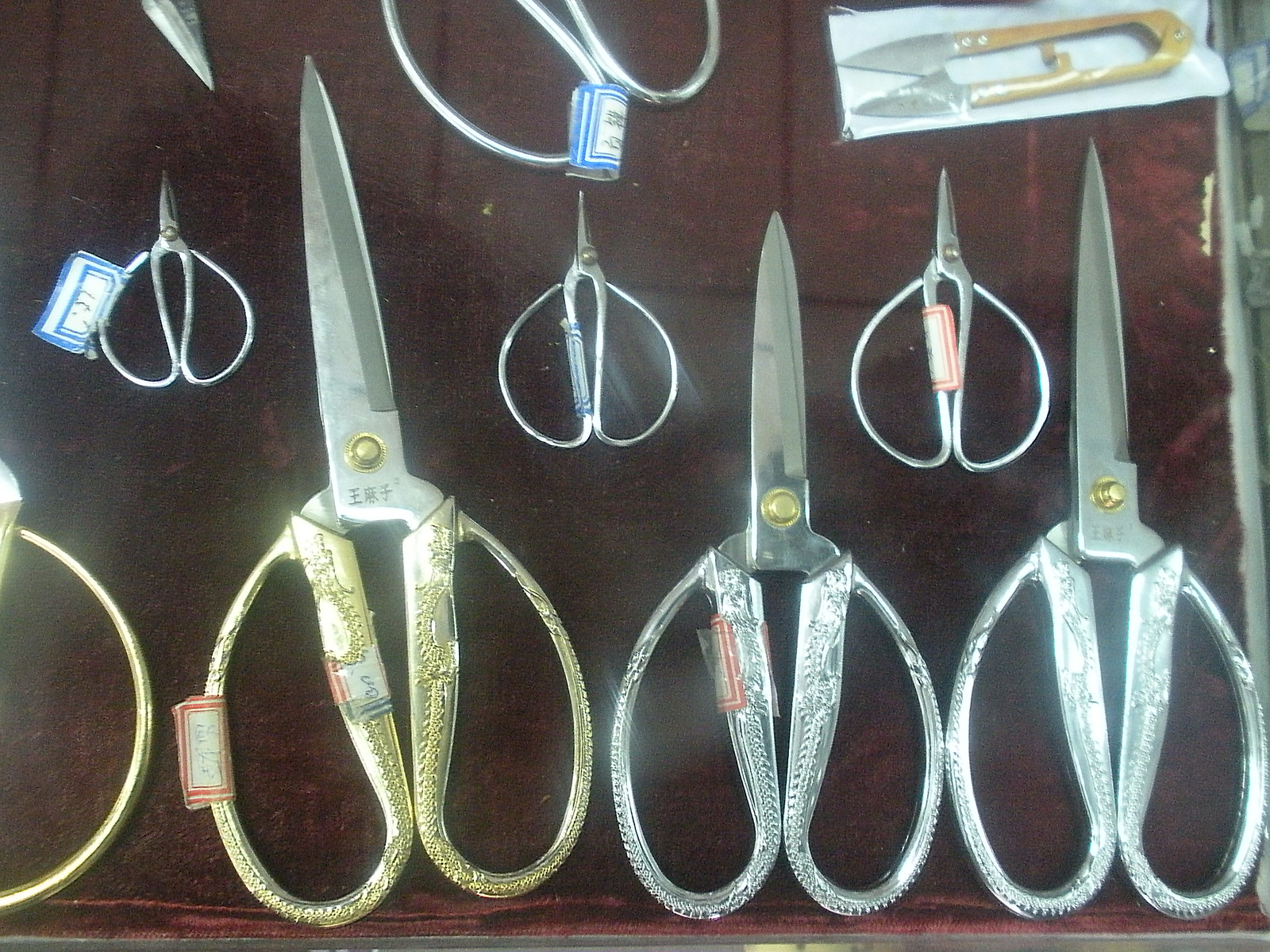This is a close-up photograph of an ornate display featuring a diverse collection of antique scissors and shears used in sewing and fabric-related crafts, set against a maroon or brownish velvet background that resembles cloth tiles, some outlined in black. Highlighted by their shiny, intricate designs, the collection includes several large silver and gold-handled pairs, embellished with detailed carvings and engraved with small letters and numbers on their blades. Three prominent, large scissors are arranged with their handles at the bottom, facing upwards. Nestled between these are smaller scissors with large handles, likely used for precision work like snipping embroidery thread. In the bottom left corner, a gold handle is visible, while the upper portions of additional ornate handles peek from the top of the image. The upper right corner features a unique tool resembling a combination of tongs and scissors, with a pewter blade and a distinctive yellow handle, contained within a small, see-through plastic pouch. The entire assortment suggests a display of both functional tools and collector’s items, emphasizing their historical and aesthetic value.